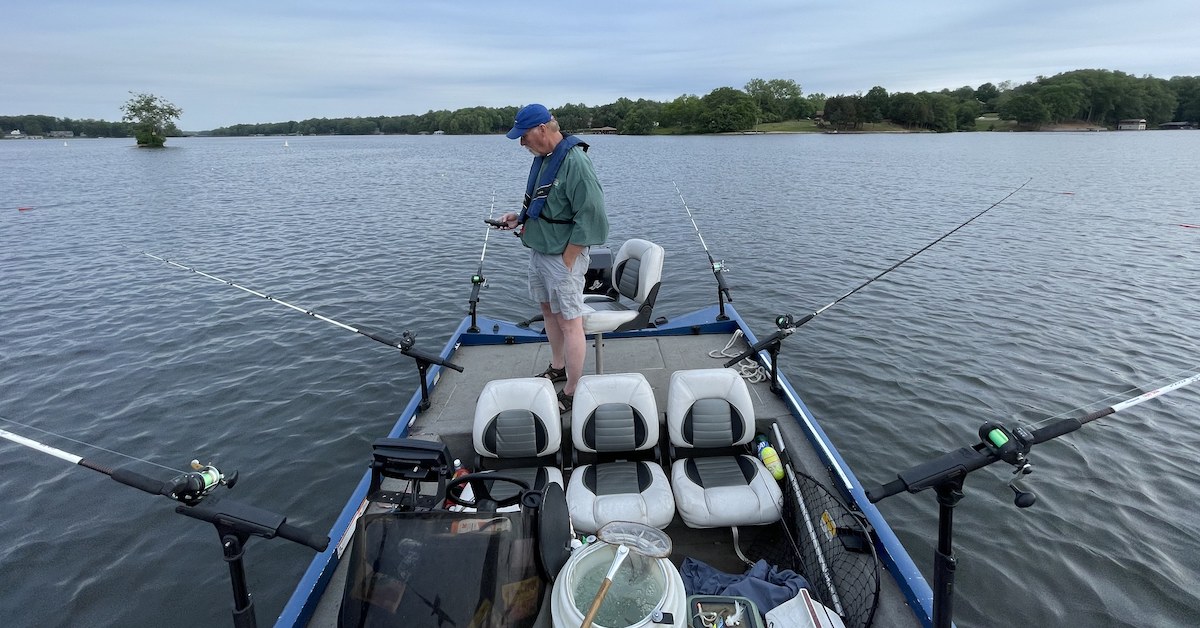The image depicts a solitary fisherman standing on a small, blue boat, situated on a lake with a backdrop of sky and distant shorelines featuring houses and minimal trees. The man, an older white individual with gray hair and a gray beard, is dressed in a blue cap, a blue life jacket tied around his waist, a dark turquoise green long-sleeved shirt, and khaki shorts. He wears black sandals and appears to be examining something on his cell phone. The boat is equipped with six fishing rods, three on each side, all set up in stands around the boat's perimeter. An upholstered white chair with black and gray sections supports the man, with three additional similar seats facing the camera. A white bucket, possibly containing ice water, is positioned in front of the middle seat, alongside a collection of fishing gear. Additionally, a net on a pole is tucked between one of the chairs and the boat's side.